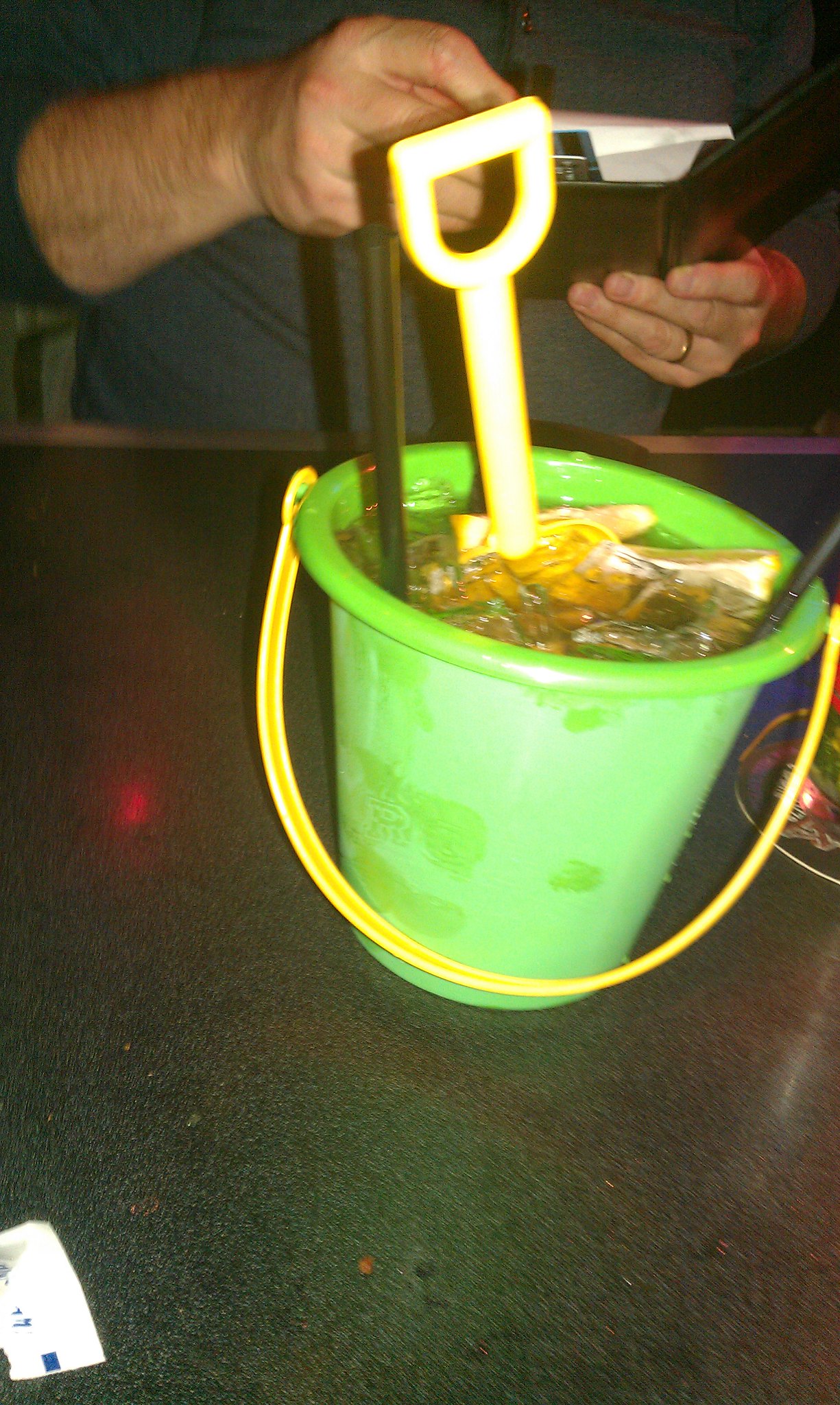The photograph depicts a small, green plastic bucket with a yellow handle, resembling those used by children at the beach. The bucket is filled with a dark beverage, ice cubes, and a yellow toy shovel. Two black plastic straws protrude from opposite sides of the drink. The bucket is resting on a black table with white and gray specks, and a small white ticket stub is visible in the bottom left corner. In the background, a man’s torso and hands are visible. He is wearing a dark gray sweater and a gold wedding ring on his left hand. He is holding a black billfold in both hands, possibly with a receipt and credit cards, indicating a restaurant setting. This style of bucket drink is reminiscent of those popular in Thailand during the Songkran water festival.